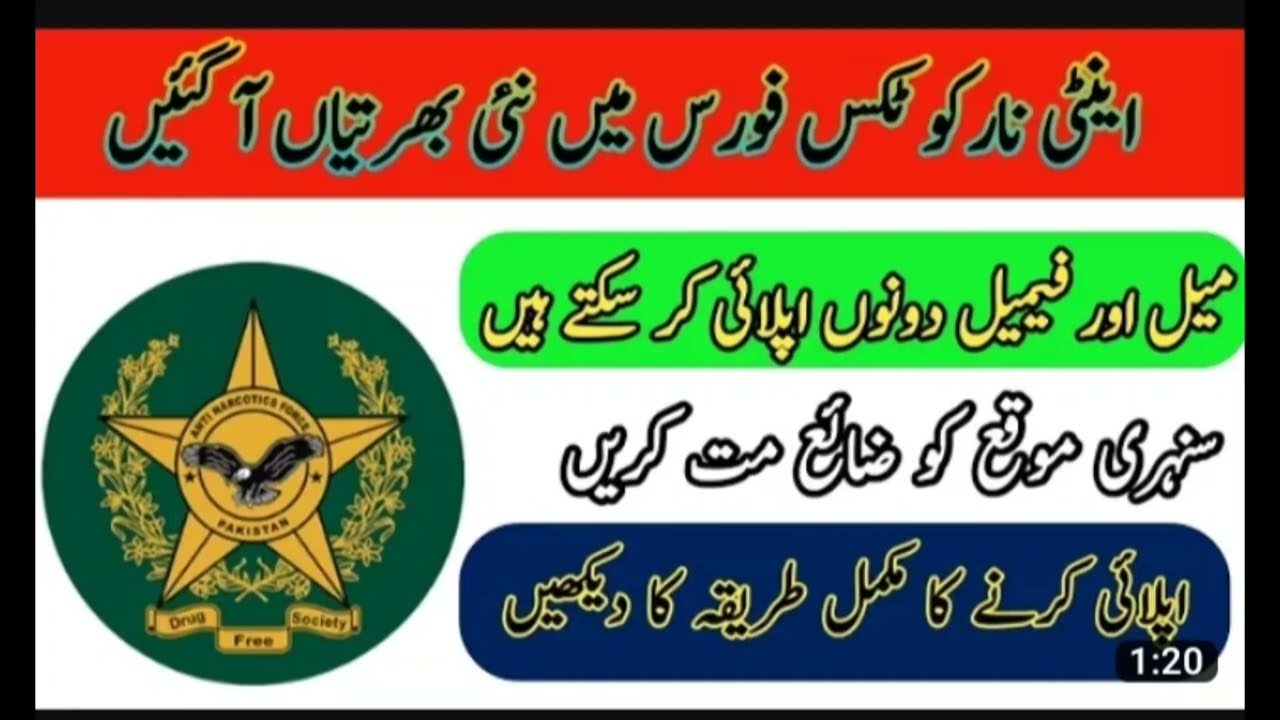The image appears to be a screen capture or a photograph of a rectangular design that resembles a flag, possibly for a company or a country. The top one-quarter of the image features a red horizontal band with foreign text in black, likely an Arabic script. Below this is a green rectangle also containing similar foreign writing in yellow. The remaining two-thirds of the background is predominantly white, displaying more of the same foreign text in black.

In the bottom right corner, there is a timestamp reading "1:20," suggesting that the image might have been taken from a video. To the left, towards the bottom, is a green circle featuring a gold five-pointed star in its center with two concentric circles inside it. An emblematic bald eagle, identifiable by its white head and flapping wings, is positioned within the star. Surrounding the eagle, the outer ring of the circle appears to feature text, though the exact wording is unclear. Below the green circle, there are three banner-like sections containing text, with the words "Drug-Free Society" being discernible.

The overall composition of the image combines elements of heraldic symbolism and structured text, creating what could be an emblematic representation or seal.